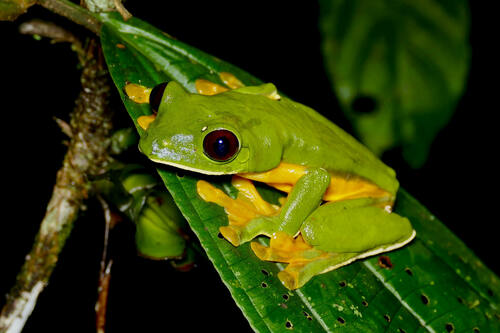In the image, a small lime green frog with a yellowish belly is perched on a large, deep green leaf with distinctive little black circles. The frog's front and back legs are the same green color, while its toes or webbing are yellow. Its bulging black eyes almost appear to have a deep red hue in the iris region. The frog is the focal point of the image, sitting on a branch diagonally extending from the left, which is brownish with a hint of white on the lower left side. Another large, fanned-out green leaf is visible in the upper right corner. The background is predominantly black, creating a stark contrast that emphasizes the frog. The scene suggests a rainforest setting, capturing a moment of wildlife in a rather dark yet natural habitat.